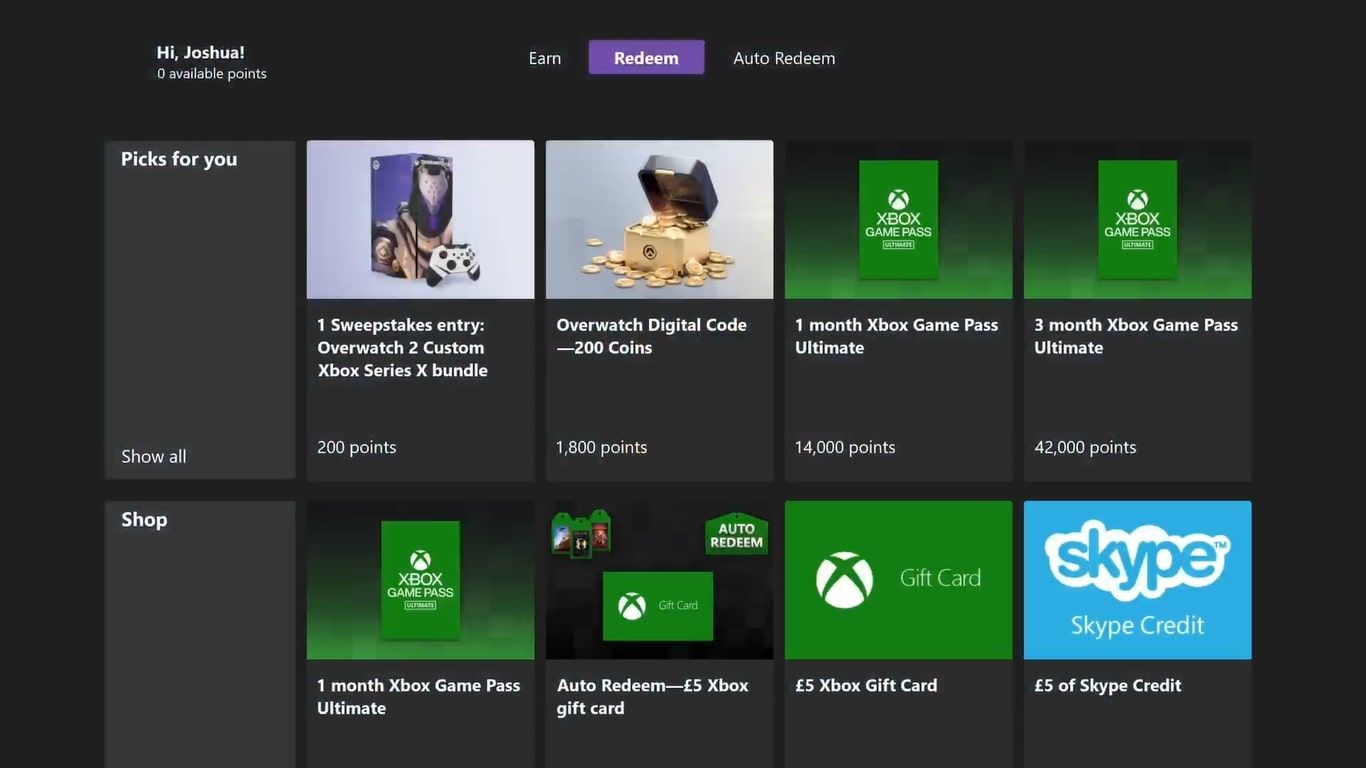The screenshot displays a section of a reward or gift card webpage set against a sleek, black background. The user, identified as Joshua by the "Hi Joshua" greeting in the upper left corner, is currently viewing the "Redeem" tab among the options "Earn," "Redeem," and "Auto Redeem," featured prominently in white font. Joshua is exploring various redemption choices available on this platform. The highlighted "Redeem" tab reveals a diverse array of options:

1. Sweepstakes Entry
2. Digital Code
3. Overwatch (for 200 coins)
4. One Xbox Game
5. 3-Month Xbox Game Pass
6. 1-Month Xbox Game Pass
7. Auto Redeem
8. 4.5 Xbox Hours
9. 65 Xbox Hours Gift Card
10. 45 Skype Credit

Each reward option is visually represented by a rectangular photo icon, illustrating the type of reward Joshua could receive. This detailed layout suggests a structured reward system tailored for gamers or individuals engaging with games. Joshua currently has approximately eight chances to claim a reward, underscoring the platform's function as a gaming-based incentive program. No additional noteworthy details are present in the screenshot.